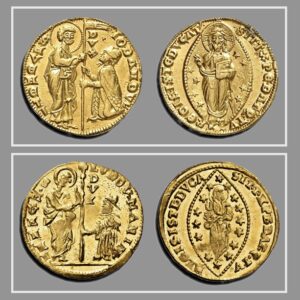The image is a staged, full-color square photograph with a gray background and a thin white border. It features four ancient-looking golden coins, arranged in two rows of two, each coin housed in its own white-bordered rectangle. 

In the top row, the left coin displays two figures: a person standing with a halo around their head, holding a staff, while another person kneels before them. The coin on the top right features a holy figure with a halo and stars around their head, holding a tablet.

The bottom row contains what appear to be lower-quality replicas of the top row's coins. The bottom left coin mirrors the top left, showing a standing figure with a halo and a kneeling person, though the design is less distinct. The bottom right coin attempts to replicate the top right but lacks clarity, with a more defined oval shape and stars around the central figure's head. The inscriptions on all coins are in a foreign language and are largely illegible due to their blurriness.